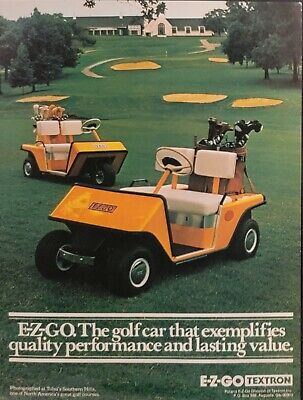This vintage-style advertisement showcases two vibrant yellow golf carts prominently positioned on a meticulously manicured golf course. The front cart, slightly angled to the left, and a second, slightly smaller cart oriented to the right, are both laden with brown golf bags and clubs. Notably, both carts lack roofs. The course features verdant green grass interspersed with yellow sand pits and a gently winding path leading up a hill. In the backdrop, a large, beige clubhouse with a black roof stands majestically, framed by scattered deciduous trees and a sliver of gray sky above. Text at the bottom of the image, bordered by bold white lines, reads, "Easy Go, the golf cart that exemplifies quality performance and lasting value," with an additional inscription, "Easy Go Textron," in the lower right-hand corner, emphasizing the brand's commitment to excellence.